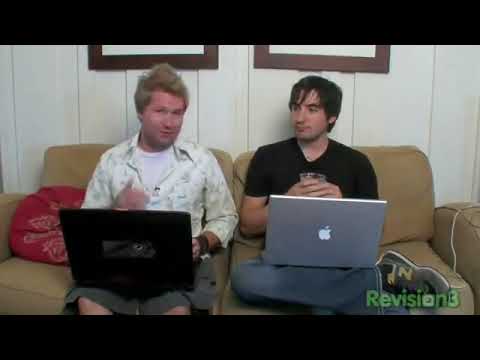The image depicts two young to middle-aged white men sitting closely together on a light tan couch against a white-paneled wall, where the bottoms of two framed pictures peek out. Both men have laptops on their laps. The man on the left is wearing a white t-shirt under a white button-down shirt with a floral pattern. He has green cargo shorts on and sports blonde hair. He is using a black laptop. The man on the right, with long black hair in a punk rocker style, is dressed in a black t-shirt, blue jeans, and New Balance sneakers with a yellow logo. He holds a cup with both hands and is working on a silver Apple laptop with a glowing white Apple logo. On the bottom right corner of the image, the green text "REVISION 3" is superimposed. A red pillow is visible in the corner of the couch, and black widescreen bars frame the image, giving it the appearance of an old video screenshot.